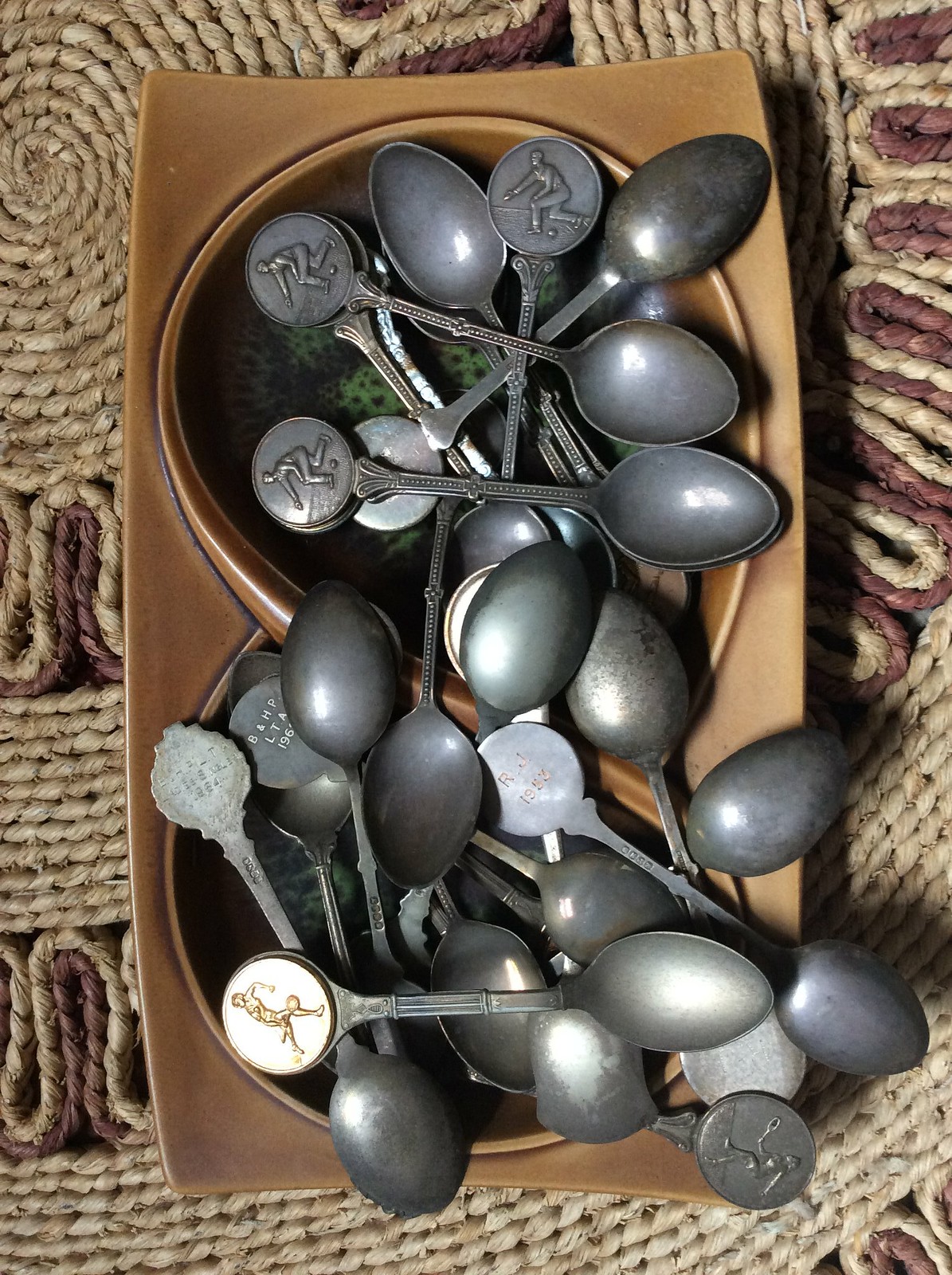This photograph showcases a collection of vintage collector's spoons, likely from the mid-20th century, displayed in a brown ceramic dish with two circular compartments. The spoons, once silver-toned, now appear tarnished and discolored with age. Each spoon features a rounded medallion at the top of the handle, depicting various sports activities such as bowling, curling, tennis, and skiing. The dish sits on a woven reed placemat, featuring light and dark brown hues. Some spoons bear engraved markings with initials and dates, including "RJ, 1953" and "BNHP LTA, 1960," enhancing the historical and collectible value of the set.